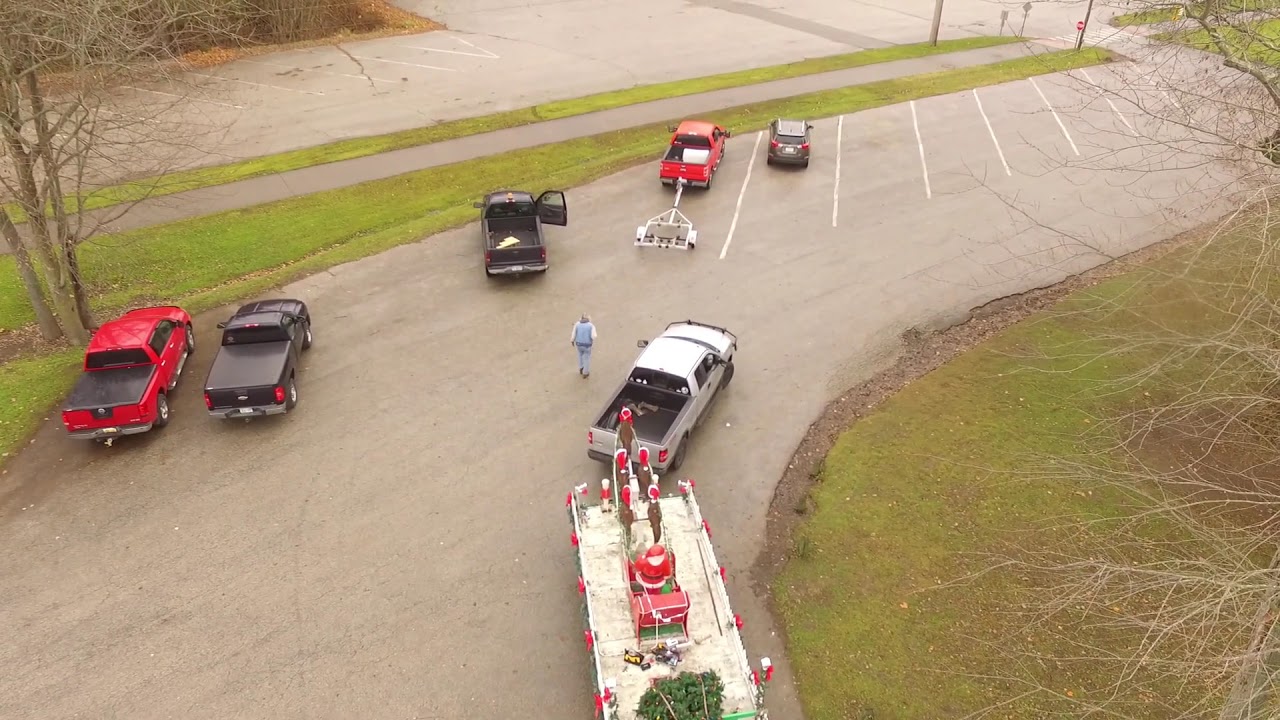This high-angle, drone-captured image vividly showcases a rectangular parking lot, possibly in winter, characterized by its nearly bare trees scattered to the left and right. Center frame features a pickup truck pulling a festive parade float adorned with Santa Claus in a red suit on a sleigh, surrounded by reindeer sporting Santa hats and decorative lights. Positioned in a smaller area of the parking lot, the truck is accompanied by a sparse presence of people, indicative of early morning parade preparations. The lot includes white-striped parking spaces, with a mix of five pickup trucks and an SUV situated predominantly on the left and center of the image. From left to right: a red pickup truck, a black one, another black truck with its passenger door open, a red truck attached to a small white trailer, and a gray SUV. More noticeable is a lone individual in a blue top and jeans walking away from the silver pickup truck and float, adding to the early setup ambiance. Additionally, the lower right side of the image features a well-maintained patch of green grass, intersected by bare tree branches and bordered by a pathway leading to more parking or a roadway.